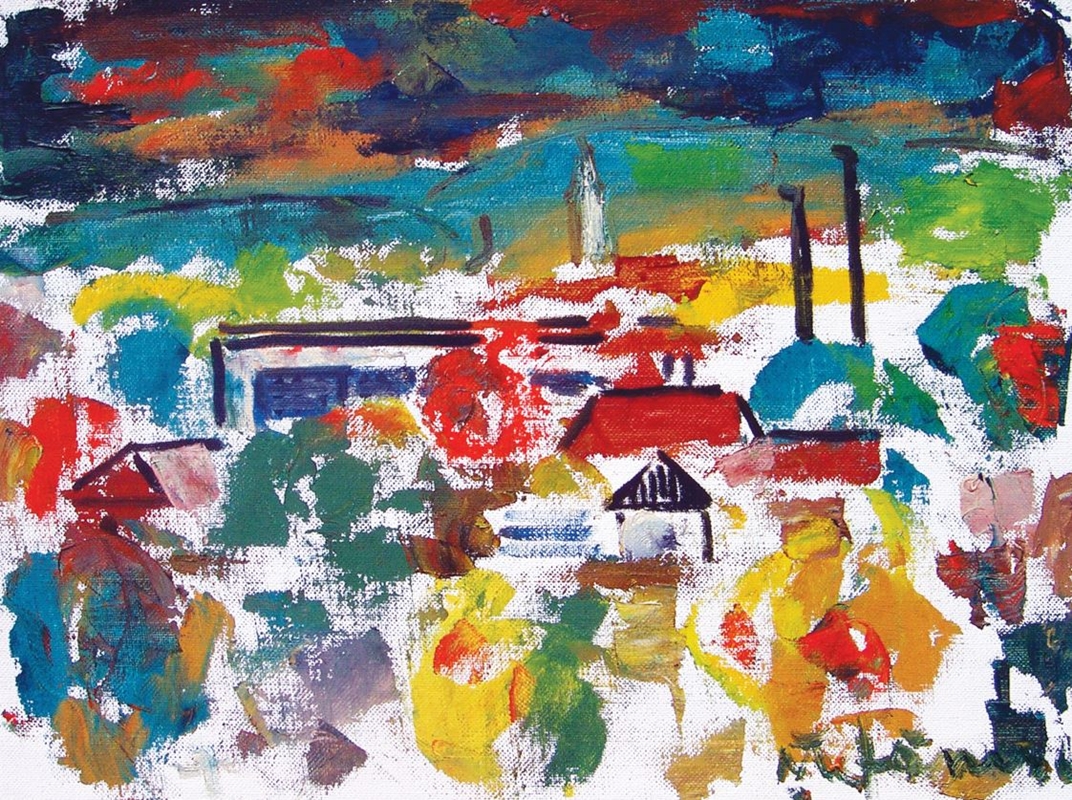This abstract painting vividly captures a bustling village from a high angle, showcasing an eclectic mix of vibrant colors. The scene is dominated by splashes of red, yellow, blue, green, and purple, creating a lively and dynamic landscape. The lower half of the artwork is filled with splotches of color that, upon closer inspection, reveal the rooftops of homes, buildings, and what appear to be factory structures with black chimneys. Some roofs are triangular in shape, painted in hues of purple and red. 

Despite its abstract nature, the painting conveys a deliberate and intricate composition, with fine, naive-like lines that subtly outline the village's architecture. Towards the center and top, there is a tall structure, possibly a steeple or a statue, that rises above the rest, adding a focal point to the composition. Above the village, green mountains and rolling hills stretch across the upper part of the canvas, interspersed with red and green shrubbery.

The sky above the village transitions to darker tones, featuring reds and purples, suggesting an evening ambiance. The painting's top section is densely colored, while the lower half reveals patches of white canvas that appear smeared, adding a raw, imperfect touch to the vibrant scene. This deliberate use of color and form creates a deceptively simple yet intricately detailed portrayal of a colorful cityscape nestled among lush hills and a dramatic sky.